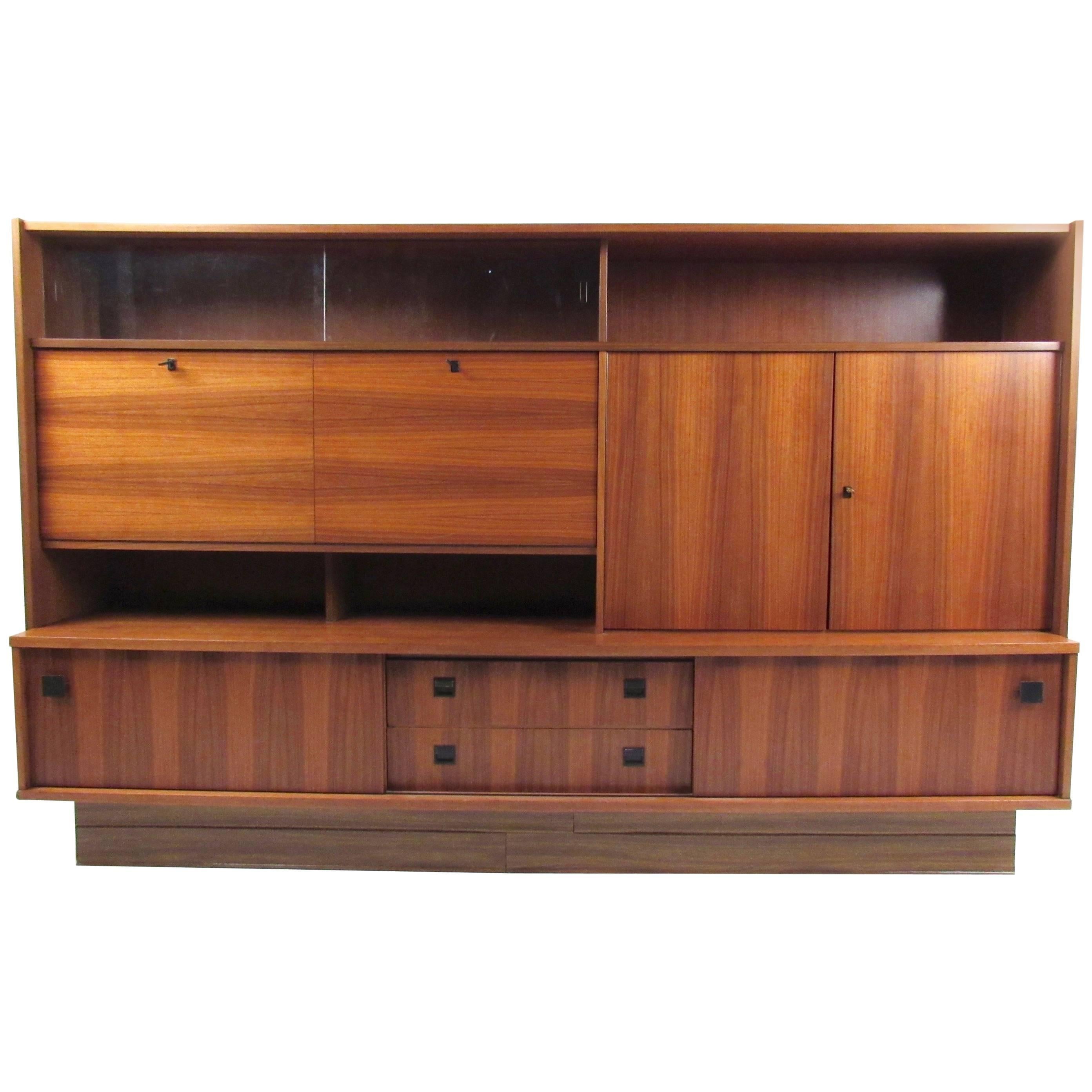This detailed image showcases an up-close view of a vintage office furniture piece, likely from the late 1950s to early 1960s. The console is predominantly made of dark mahogany wood with a rusty patina, adding to its aged appearance. The top left corner features glass panels with handles for access, while the far right side has an open section without glass, equipped with a small drawer and a handle for easy retrieval. Below, on the bottom left, another compartment with a handle can be pulled open, adjacent to two drawers accessible from either side. The entire setup is characterized by its modular and square design, featuring varying wood grains and sliding panels typical of mid-century modern aesthetics. Standing at a couple of feet tall, this console is reminiscent of a storage cabinet wall unit, possibly used for holding a television or records, embodying the functional simplicity and angular design iconic to that era. The photograph is set against a plain white background, highlighting the unit's architectural lines and clear divisions among its shelves and storage areas.